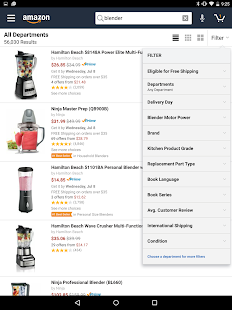The image is a screenshot of the Amazon application displayed on a smartphone. At the top, the phone's status bar indicates that Wi-Fi is enabled, the battery is at approximately 35% charge, the time is 9:25, and Bluetooth is enabled. 

The upper section of the Amazon app features a dark blue banner with the recognizable white Amazon logo alongside the yellow arrow. Directly below, there is a search bar, a microphone icon, and a cart icon showing one item. The search query entered is "kitchen appliances for blenders," which yielded 56,220 results, spanning all departments. 

A filter menu has appeared with options including eligible for free shipping, departments, delivery day, brand, condition, and average customer review. 

Displayed are several blender options, such as a Hamilton Beach blender priced at $25, characterized by its black and silver color scheme. Additionally, there is a smaller, less expensive blender priced at $14.95.